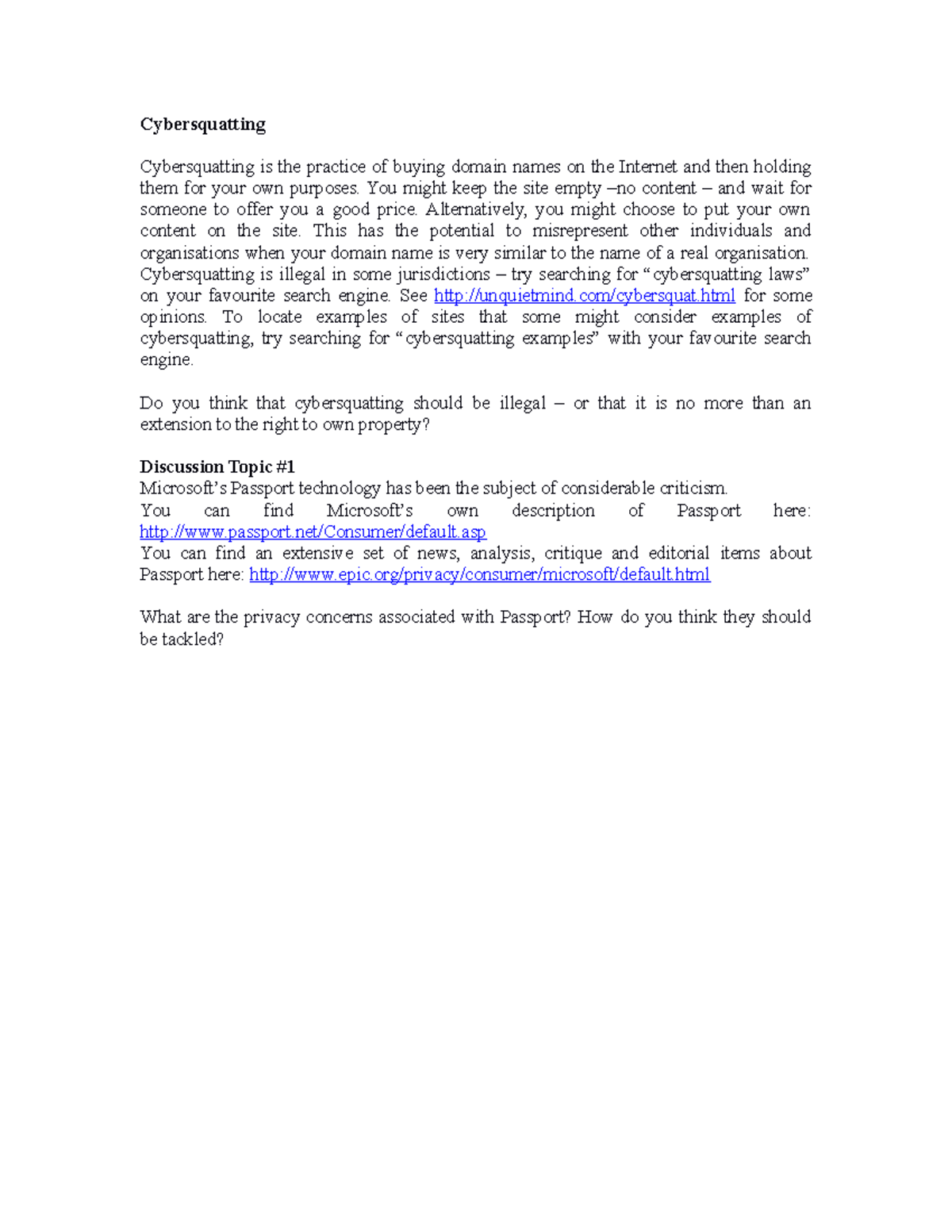This image contains a detailed explanation of the term "cyber squatting." It defines cyber squatting as the practice of purchasing domain names on the internet and holding onto them either for personal use or to sell them at a significant profit later. The description notes that cyber squatters might leave these domains empty, devoid of content, while waiting for potential buyers to make lucrative offers. In other cases, they might populate the site with their own content, which can lead to the misrepresentation of other individuals and organizations, especially when the domain name closely resembles that of an established entity. The text highlights that cyber squatting is illegal in certain jurisdictions and encourages readers to research cyber squatting laws using their preferred search engine. Additionally, there is a link provided for users to explore various opinions and locate specific examples of what some might consider instances of cyber squatting by conducting an online search for "cyber squatting examples." The description continues beyond this point.